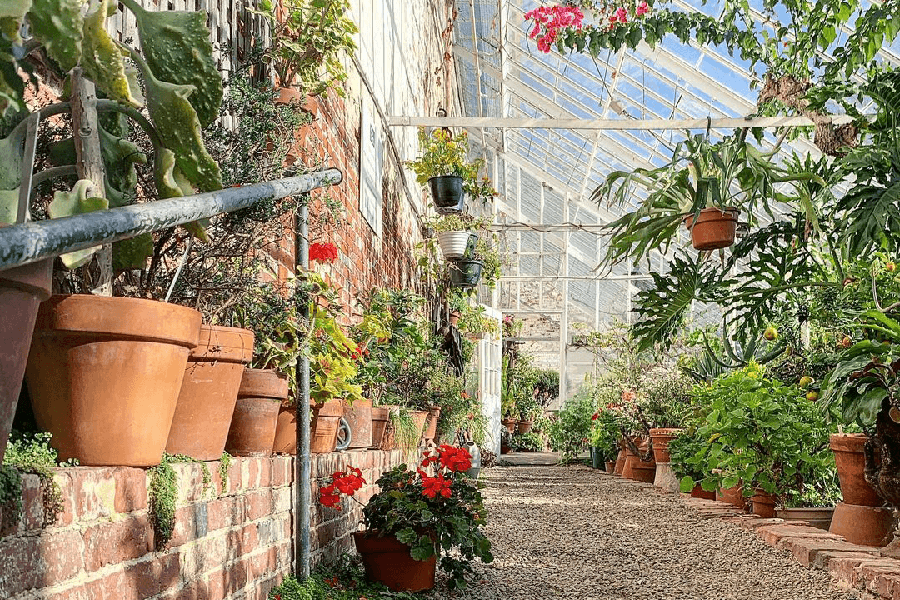This captivating image depicts the interior of a sprawling greenhouse, seamlessly attached to the side of a house. The left side of the picture showcases a red brick wall from the house, adorned with a ledge that holds an array of clay pots brimming with verdant foliage, including geraniums. Some of these clay pots hang from the roof, which is made of glass set in a sturdy metal frame. A gravel walkway runs parallel to the house, leading the viewer's eye deeper into the greenhouse, hinting at more sections to explore. On the right side of the image, against the backdrop of the slanted glass roof that extends downwards at a 45-degree angle, additional clay pots and green plants are neatly lined up. Pink blossoms from what appears to be an overhanging tree add a splash of color, enhancing the serene and tranquil ambiance. The glass wall at the rear of the greenhouse features a door, inviting further exploration and underlining the greenhouse’s spaciousness and thoughtfully designed layout.